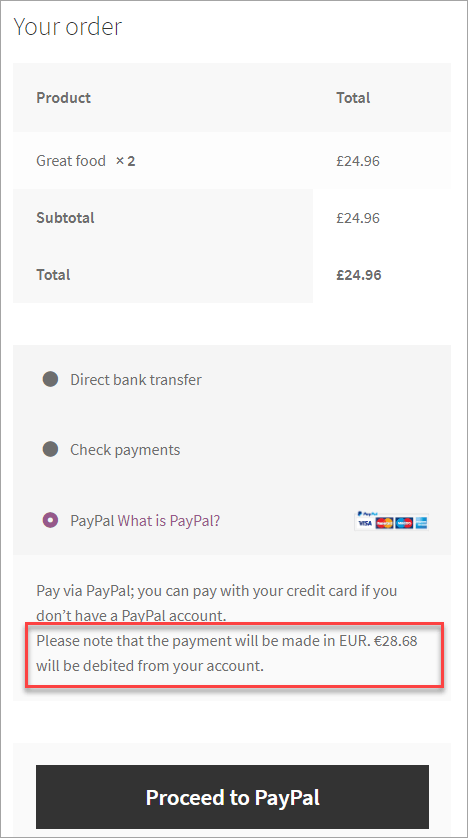This vertically oriented mobile phone screenshot depicts an order page with detailed payment options. At the top left corner, thin gray text reads "Your Order," followed by a section labeled "Product" on the left side. Directly below, it lists "Great Food × 2," alongside corresponding costs. The subtotal and total both amount to £24.96.

Beneath this section is a light gray outlined box containing three bullet points. The first point lists "Direct Bank Transfer," the second is "Check Payments," and the third, highlighted in purple and featuring a white circle, indicates "PayPal." Accompanying this are icons for PayPal, Visa, MasterCard, and American Express.

Following this, there's text that reads, "Pay via PayPal. You can pay with your credit card if you don't have a PayPal account." Highlighted in a red box below is a notice stating, "Please note that the payment will be made in EUR. $28.68 will be debited from your account."

At the bottom of the image, a black horizontally oriented rectangular button with white text prompts, "Proceed to PayPal."